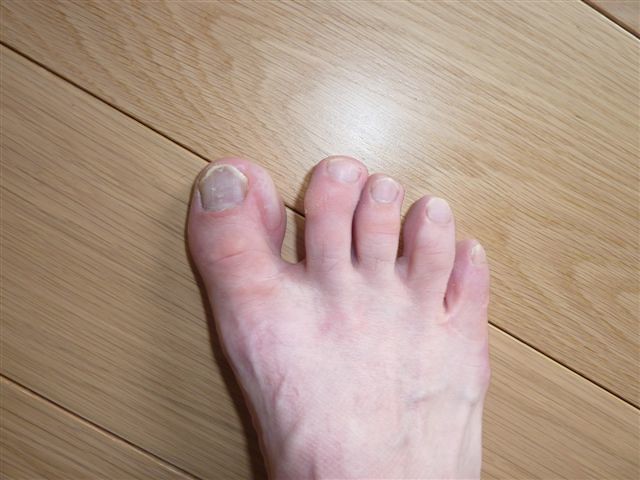This is a detailed, wide rectangular image capturing a white-skinned foot positioned flat on a light brown, diagonally paneled wooden floor. The foot is photographed from above, halfway visible with all toes centered in the frame. The wooden panels run diagonally from the top left to the bottom right of the image, reflecting indoor lighting that highlights the tan color of the floor. The big toe, positioned to the left, is slightly extended outward, away from the other four toes which are curled in the opposite direction. The toenails are opaque and appear to be trimmed short. Notably, the big toe exhibits signs of an infection: a red inflamed area is visible to the right of the nail, with a pale, somewhat inflated portion on top. The overall setting and lighting suggest an indoor environment.